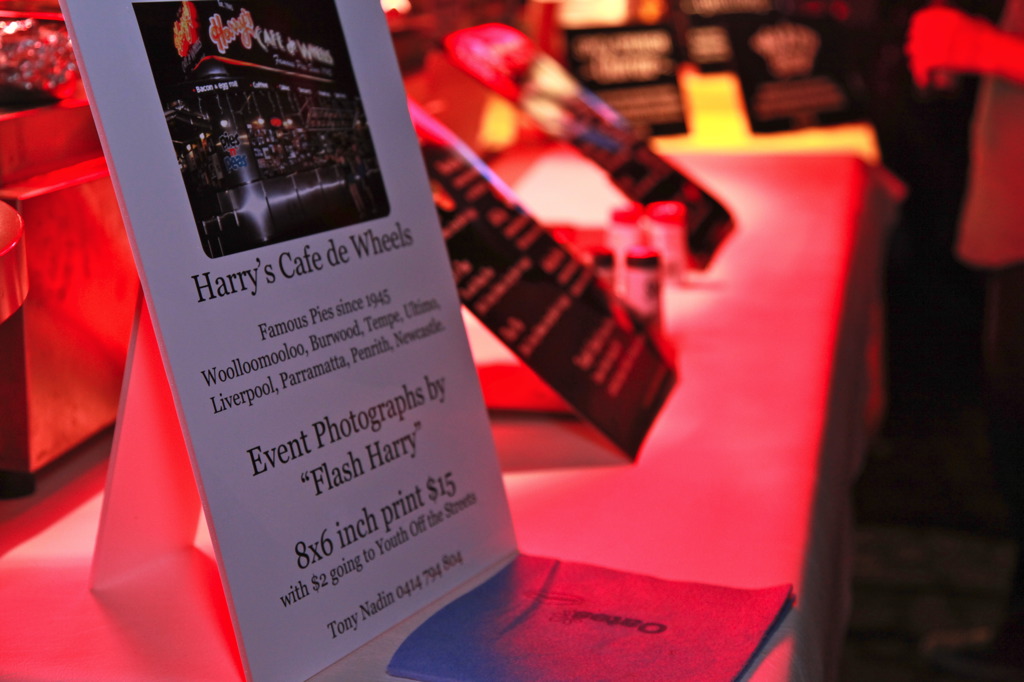The image depicts a table draped with a white tablecloth, illuminated by a red spotlight, creating a predominantly red and white-blue color scheme. Centered on the table are several 8x6 inch placards, leaning upright. The most prominent placard features a white background with black text and a photograph of a building, identified as Harry's Café de Wheels. The text under the photograph reads: "Harry's Café de Wheels, Famous Pies Since 1945." Listed below are multiple locations including Woolloomooloo, Burwood, Tempe, Ultimo, Liverpool, Parramatta, and Penrith. Additional text indicates that event photographs by Flash Harry are available, with prints priced at $15, of which $2 goes to 'Youth Off The Streets.' The contact details, Tony Naden, and phone number, 0414796804, are noted at the bottom. In the background, several people can be seen reading the placards, further contributing to the detailed setting.